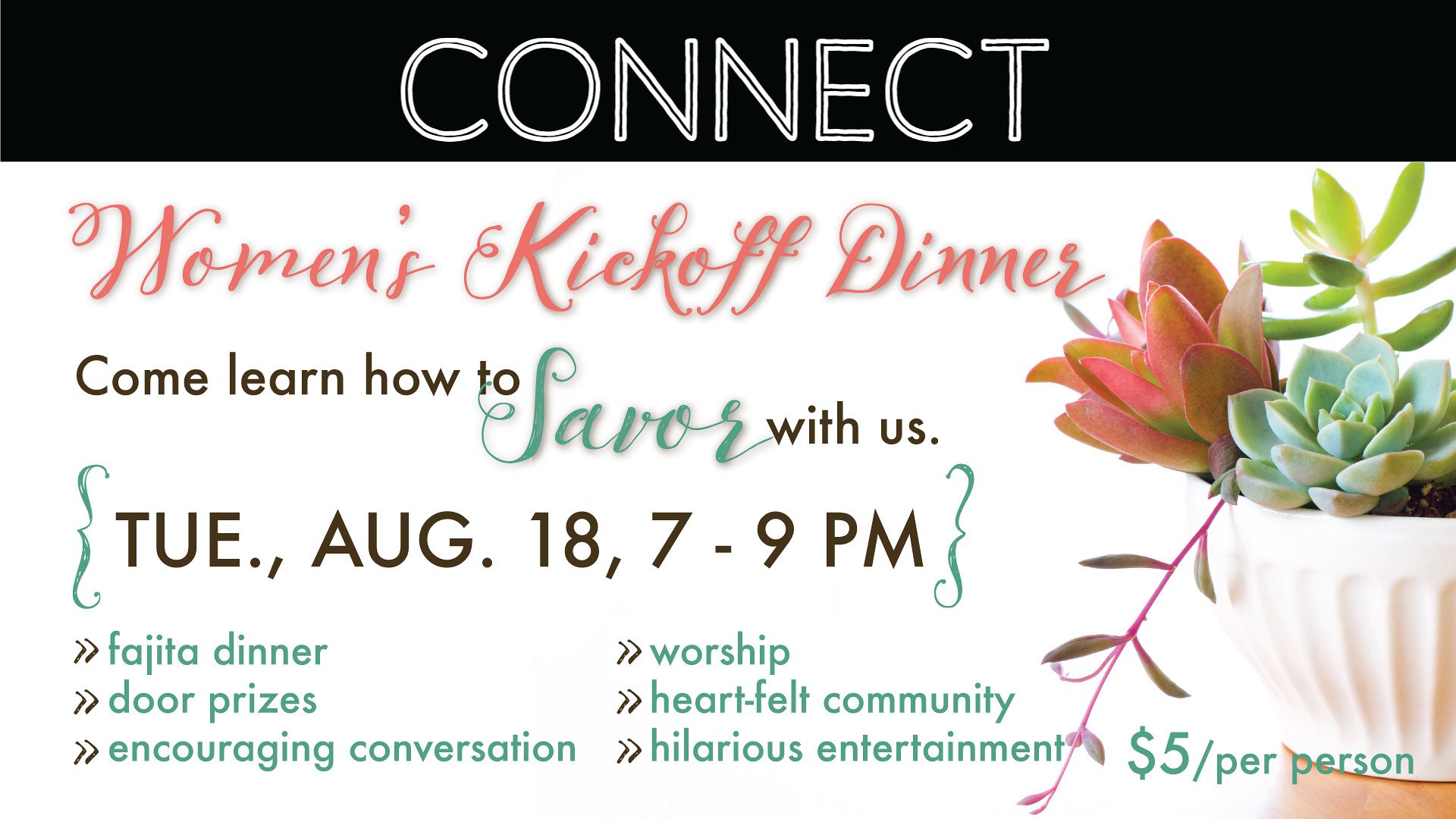This image is a digital advertisement shaped like a high-definition TV screen. At the top, there is a black band with the word "Connect" written in large, white letters, each of which is crossed by a black line. Beneath this is a section with a white background featuring the pink, cursive text "Women's Kickoff Dinner," accompanied by a nearby image of a white planter holding desert plants. Further down, the text reads, "Come learn how to savor with us," with the word "savor" styled in green cursive. In black text, it details the event date and time: "Tuesday, August 18th, 7 to 9 p.m." Towards the bottom, in the same green color as "savor," the advertisement lists event highlights such as "fajita dinners," "door prizes," "encouraging conversation," "worship," "heartfelt community," and "hilarious entertainment." On the bottom right corner, it states "$5 per person" in green text.